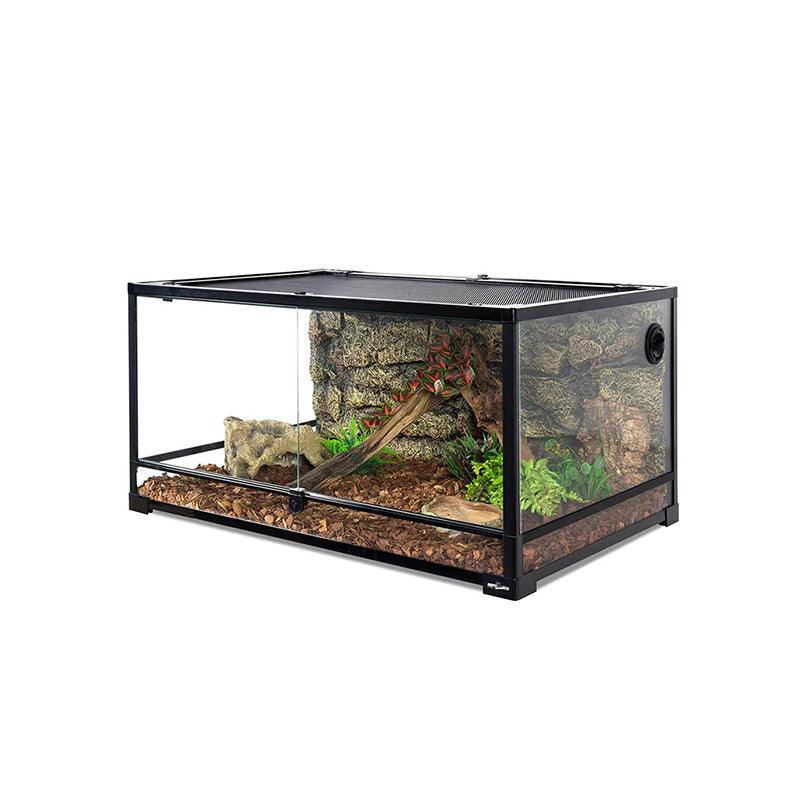The image depicts a large glass terrarium, reminiscent of a 40-gallon fish tank but distinguished by its wrought black metal frame and glass panels. The top is crafted from black metal mesh, providing ventilation. Inside, the habitat exudes a tropical ambiance, featuring a prominent grey stone rock wall at the back. The terrarium floor is lined with dark brown or cedar-colored wood chips. Lush green ferns and a few strategically placed rocks contribute to the naturalistic setting. A striking piece of ivy, showcasing vibrant green and red hues, adds a pop of color. On the left side of the tank, there is a rock habitat, while the right side houses a water dish designed to resemble a tree stump. The enclosure is accessible via two glass panels that swing forward, secured by a padlock. No animals are currently visible within the terrarium.